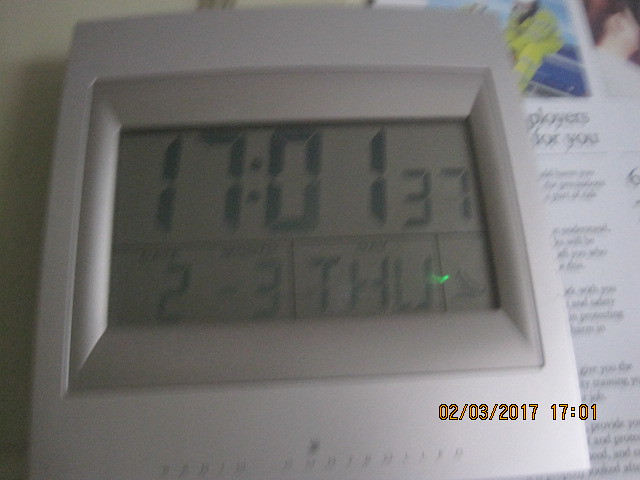This is an overhead shot of a digital clock with a white body and a silver-framed face. The display shows precise digital numbers indicating the time as 17:01:37 (5:01:37 PM). Below the time, two rectangular sections provide additional information: the month, day, and day of the week. The date displayed is Thursday, March 2nd. Based on the timestamp at the bottom of the clock display, this image was taken on March 2, 2017, at 17:01.